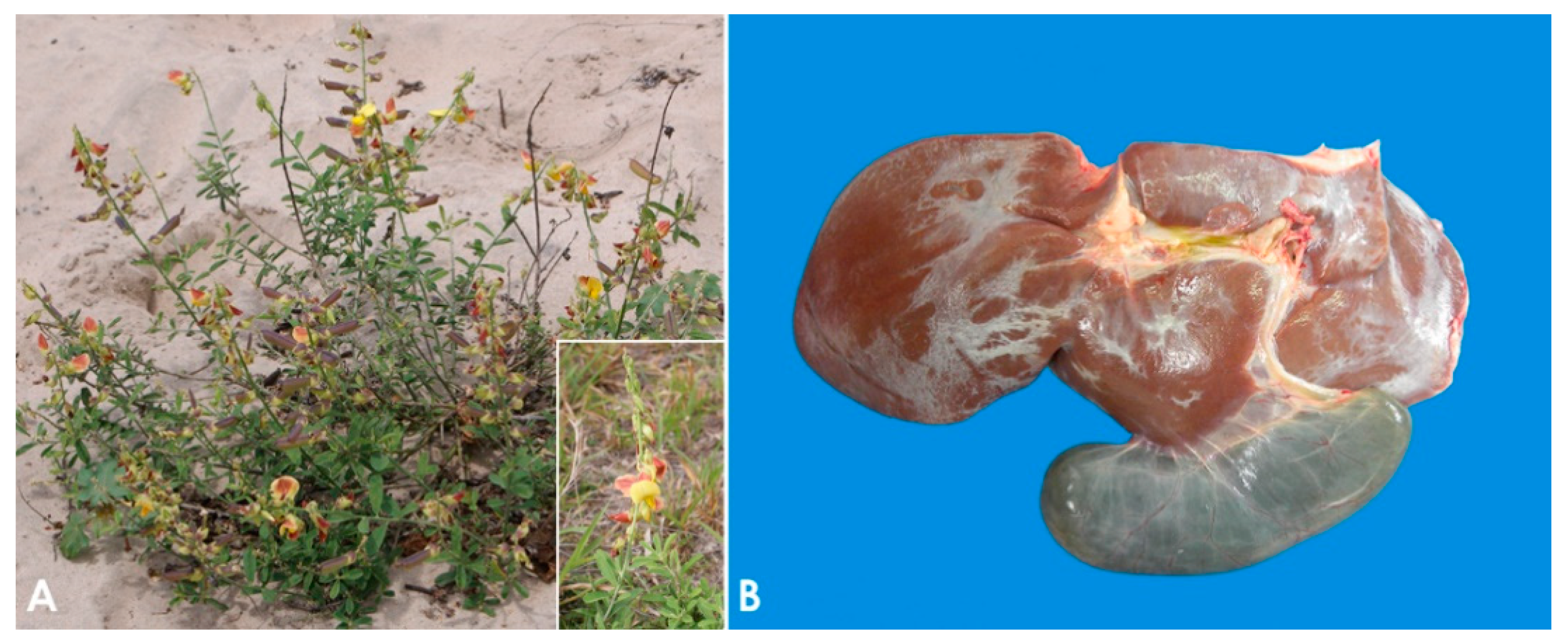The image is divided into two sections labeled A and B. 

**Image A**: This section features a photograph of a plant set in a substrate resembling either beach or desert sand. The lighting suggests it was taken either in the shade or near sunset, providing a soft, diffuse light with no harsh shadows. The plant is characterized by several upright stalks sprouting from the sandy ground, each adorned with small green leaves. Toward the top of some stalks, vibrant yellow and orange flowers are in bloom. In the bottom right corner of Image A, there is an inset close-up highlighting one of these flowers in greater detail.

**Image B**: The adjacent section presents an image against a strikingly bright blue background. It displays an organ that appears to have been surgically removed from a body. The exact nature of the organ is ambiguous, but it possesses a shape and texture that could suggest either a kidney or liver, though the latter seems more plausible upon closer inspection.